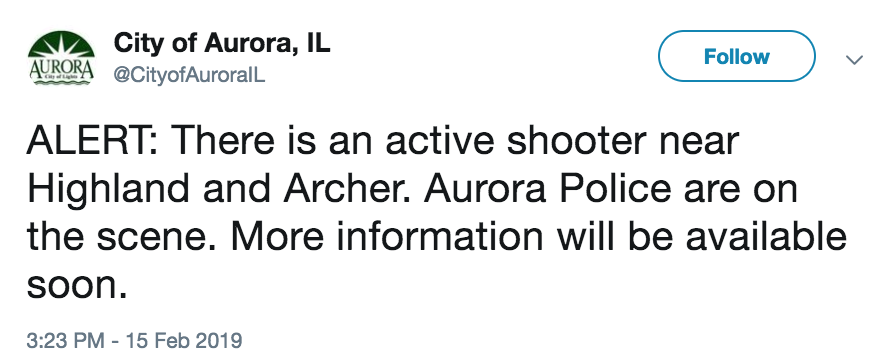This is an image of a tweet from the social media platform X, formerly known as Twitter, originating from the City of Aurora, Illinois. At the top-left corner of the tweet, there is a symbol of the City of Aurora followed by the text, “City of Aurora, IL.” Below this, the tweet text begins with an urgent alert which states: “Alert: There is an active shooter near Highland and Archer. Aurora police are on the scene. More information will be available soon.” The tweet is timestamped at 3:23 p.m. on February 15th, 2019. To the right side of the tweet, there is a blue-outlined button labeled "Follow."